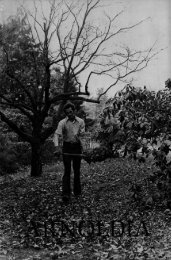This is a tiny, somewhat unclear black-and-white photograph of a man standing in a garden-like area, possibly his yard. The man, who has very short hair, is positioned in the center of the image, surrounded by a grassy area covered with leaves. He is wearing long black pants and a long-sleeved white shirt. The photo is somewhat dark, suggesting a gray sky, and the image is not very sharp. To his left, there stands a large bare tree with no branches, contrasting with the very tall, full, leafy trees in the background. On the right side of the picture, additional full trees and bushes are visible. A large bush is situated prominently in the foreground to the right. The man appears to be making a gesture, possibly throwing seeds on the ground, though it's hard to tell for sure due to the image's lack of clarity. There are also some details of flowers with tall white petals and green stems nearby. At the bottom of the tiny photograph, black letters are present, though they are difficult to make out. In the far background, just beyond the trees, a house can be faintly seen.